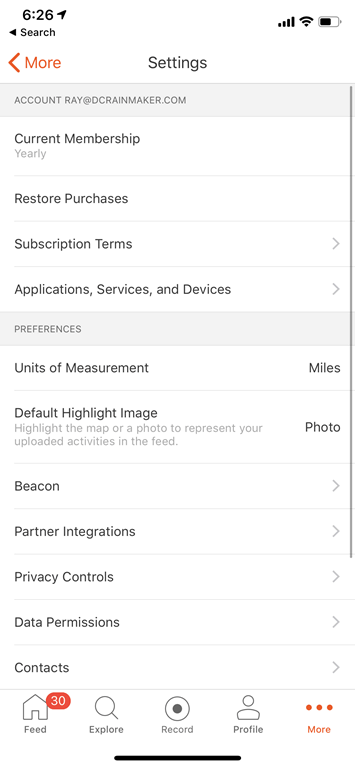This image is a screenshot of a cell phone settings screen with a timestamp of 6:26 displayed in the top left corner. The upper right corner shows icons indicating full cell phone reception, full Wi-Fi strength, and a battery level at approximately 50%. 

Below the status indicators, the settings menu is visible. At the top of this menu, a gray bar displays the account information: rayatdcraymaker.com. Under this account information, it specifies the current membership type as "yearly."

Following this, there is an option labeled "Restore Purchases." Further down, there’s a section titled "Subscription Terms," accompanied by a right-pointing arrow, suggesting additional options or information. 

Next, there is a header labeled "Application Services and Devices," also with a right-pointing arrow for further details. 

Moving down the menu, in the section named "Preferences," the units of measurement are set to miles, and the default highlight image setting is a photo. 

Finally, the menu includes options for "Beacon," "Partner Integrations," and "Privacy Controls."